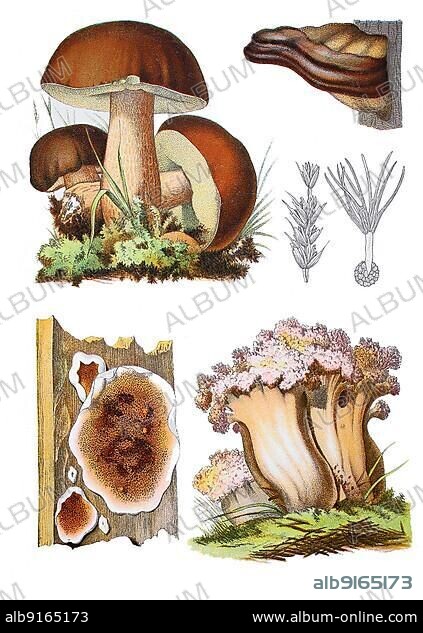Illustration of various types of mushrooms created using ink and colored with markers, paint, or possibly colored pencils. The mushrooms predominantly feature shades of brown and beige, with some green accents. The illustration includes four different types of mushrooms, with two growing out of the ground and two growing from wood. In the background, there are detailed black and white sketches of plant-like forms, including lichen. The image is overlaid with a faint gray watermark that says "Album." Along the bottom, there is a black rectangle containing white text that reads "www.album-online.com" and "ALB9165173."